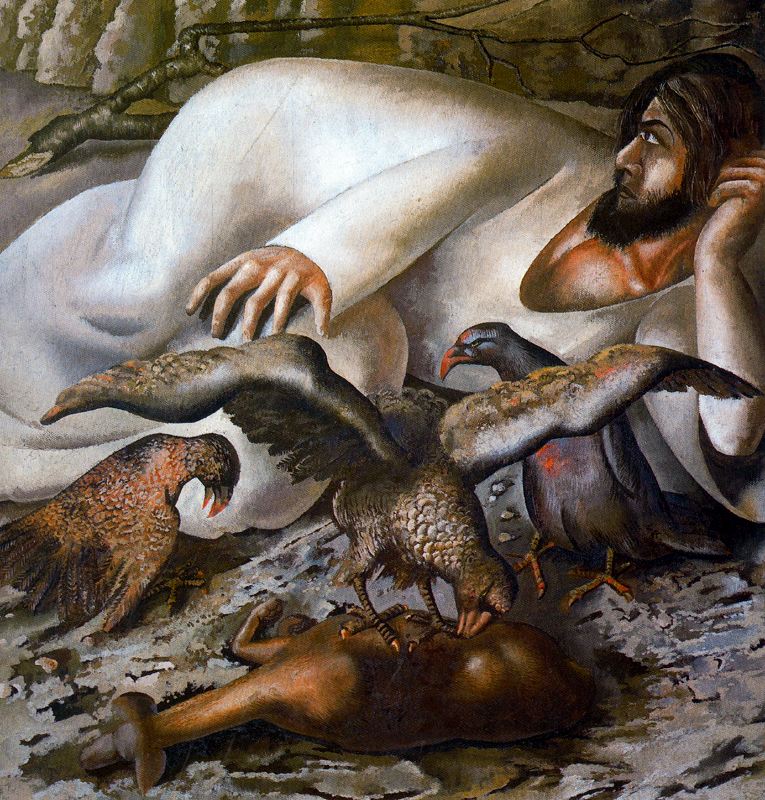The painting titled "Christ in the Wilderness, the Eagles" by Stanley Spencer, created in 1943, is a neo-Romantic work depicting Jesus lying on his side, dressed in a long white garment with a V-neck that reveals part of his chest. His black hair and long beard frame his contemplative face as he gazes off to the side. The background suggests a cave with a rocky and grayish, silvery brown ground, along with a fallen branch and scattered rocks. Dominating the lower foreground are three birds, dark in color—blacks and grays—with large, curved beaks resembling ravens or vultures. These birds are feasting on the carcass of a dead animal, possibly a dog or another bird, adding a sense of chaos and morbid activity to the scene. Despite the title referencing eagles, the birds' characteristics align more with ravens or vultures, contributing to the painting's somber and contemplative atmosphere.